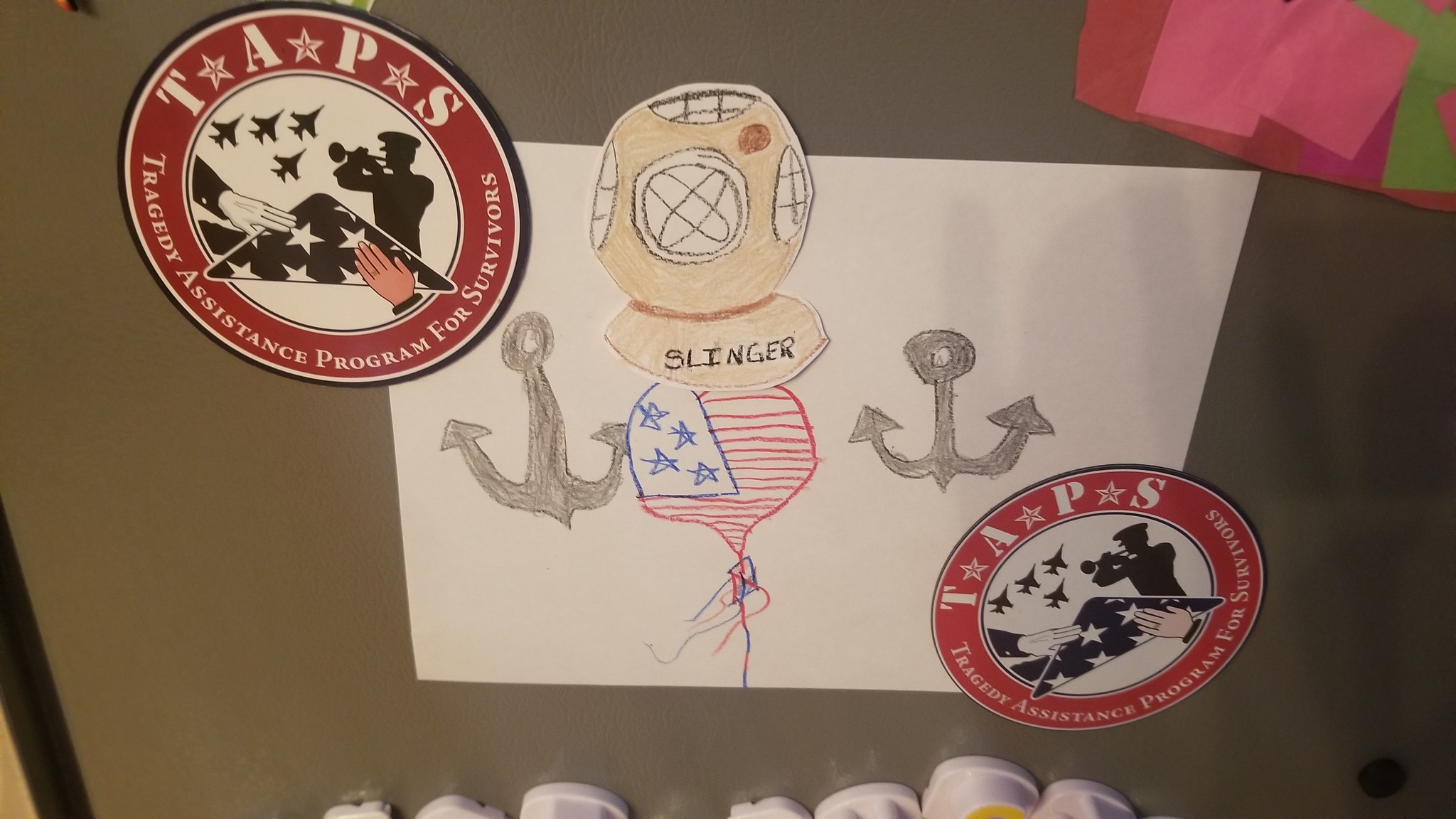A drawing or colored sheet is affixed to a flat gray metal surface, likely a refrigerator, using two round magnets. The magnets are white with red borders and feature the letters "TAPS" in white on the red border, standing for "Tragedy Assistance Program for Survivors." Inside the white circle of the border is a depiction of a folded black flag adorned with white stars, symbolizing a military folded flag. Surrounding the flag are small silhouettes of fighter jets, and to the side, there are two hands: one depicted in a light peach skin tone and the other in stark black and white. Behind the flag, there is a silhouette of a figure wearing a military-style cap, solemnly playing a bugle. The overall image resonates with themes of military service and remembrance.